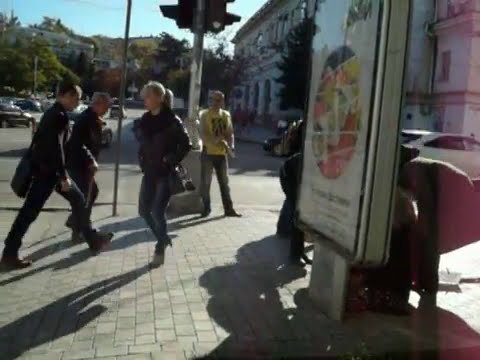The image depicts a bustling cityscape at a traffic intersection, likely in a suburb or large town. The foreground features a cobblestone sidewalk with a sign that could be a bus stop or bench, though the details are unclear. The sign also seems to advertise a plate of food. Just beyond the sign, a traffic post with a partially visible light is present. To the left, a street populated with several cars extends into the background, flanked on the right by a long, white stone building. This building lies behind a large walkway bustling with activity. There are five indistinct figures—one woman and three men, their ages ranging from early 20s to mid-50s or 60s—walking around. Among them, a young man in a yellow shirt seems to be holding or selling something. The setting appears to be outdoors in a public area, possibly downtown, with the sun casting long shadows, suggesting early morning or mid-day. The scene is colored in a palette including black, brown, yellow, gray, red, pink, purple, light blue, and tan.